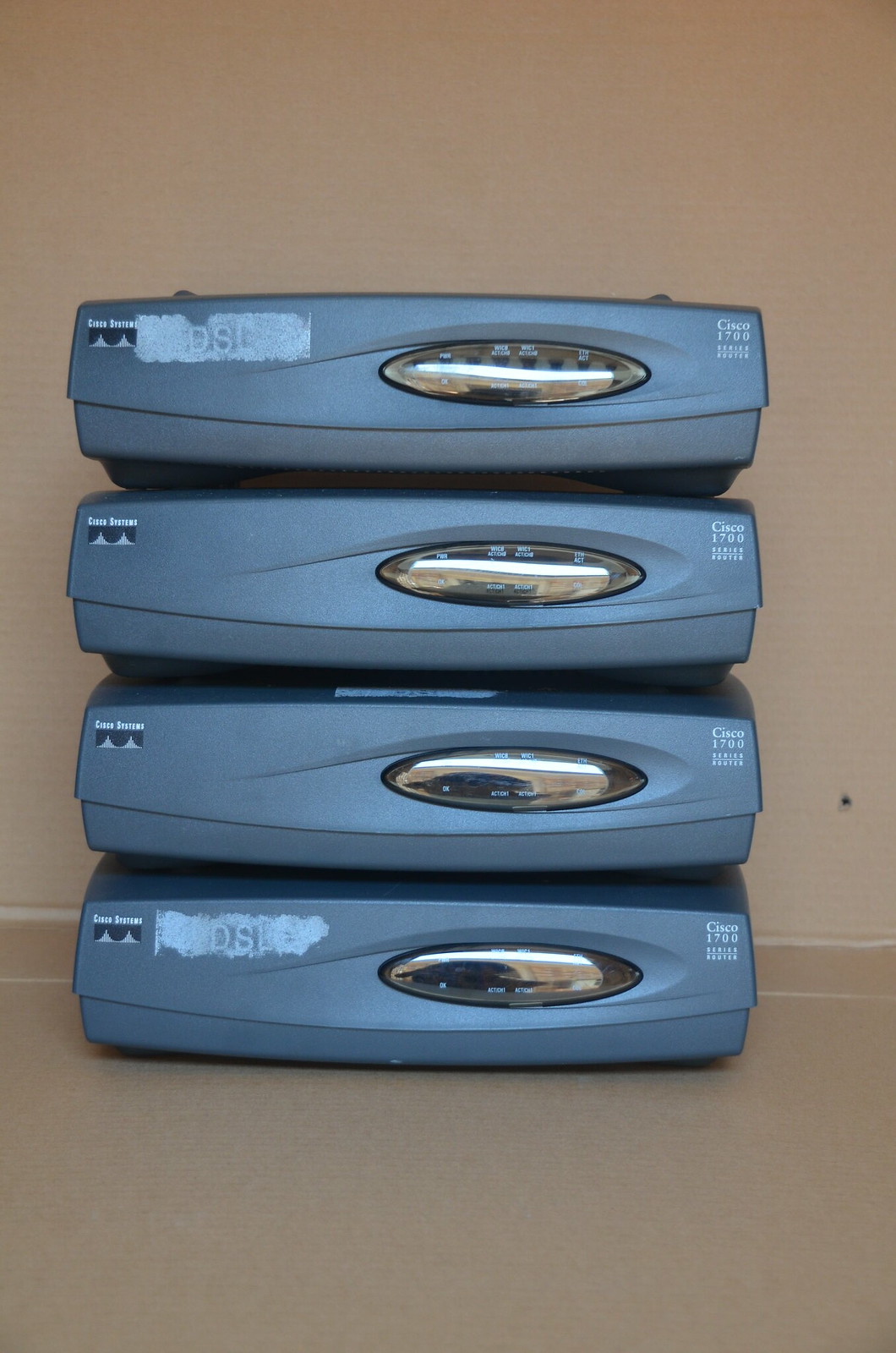The image displays four old-timey blue cable boxes stacked vertically on a tan table with a lighter tan background that fades to gray in the center. Each box features round, silver oval panels on the front, adorned with small diagrams and labels such as "volume up" and "channel number." The boxes also have logos located in the top right and top left corners. The portrait-oriented image captures a faint text, possibly "Canon," and some indistinguishable letters like "OS" or "DS." An additional blue material is visible between the second and third boxes. Despite the glare on the silver panels, every box appears identical with thick and sturdy builds.